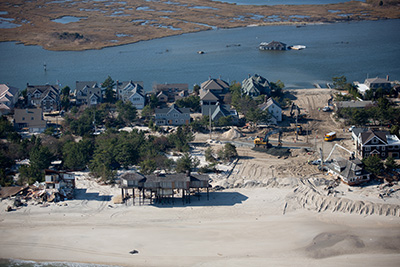This high-altitude, landscape-oriented photograph captures a scenic seaside village situated by a dark blue body of water. The village is positioned between two expansive bodies of water, giving it a peninsula-like appearance. The houses along the beach predominantly feature a two-story design with blue siding and triangular brown roofs. Interspersed among these are bungalows perched on tall stilts, surrounded by a lot of white sand. 

In the center of the image, there is noticeable construction activity with trucks and equipment visible, surrounded by patches of green trees and segmented by roads, one of which has a school bus on it. Toward the lower portion of the picture, more bungalows on stilts are visible, emphasizing the beachside setting. In the water towards the upper right of the image, there appears to be a partially submerged house or perhaps a boat, adding intrigue to the scene.

At the very top of the image, there are patchy areas of swampy terrain, possibly mangroves, characterized by green patches intermixed with the blue waters. This northern locale, evidenced by glimpses of snow around the village, highlights the unique blend of residential life, natural beauty, and ongoing development.